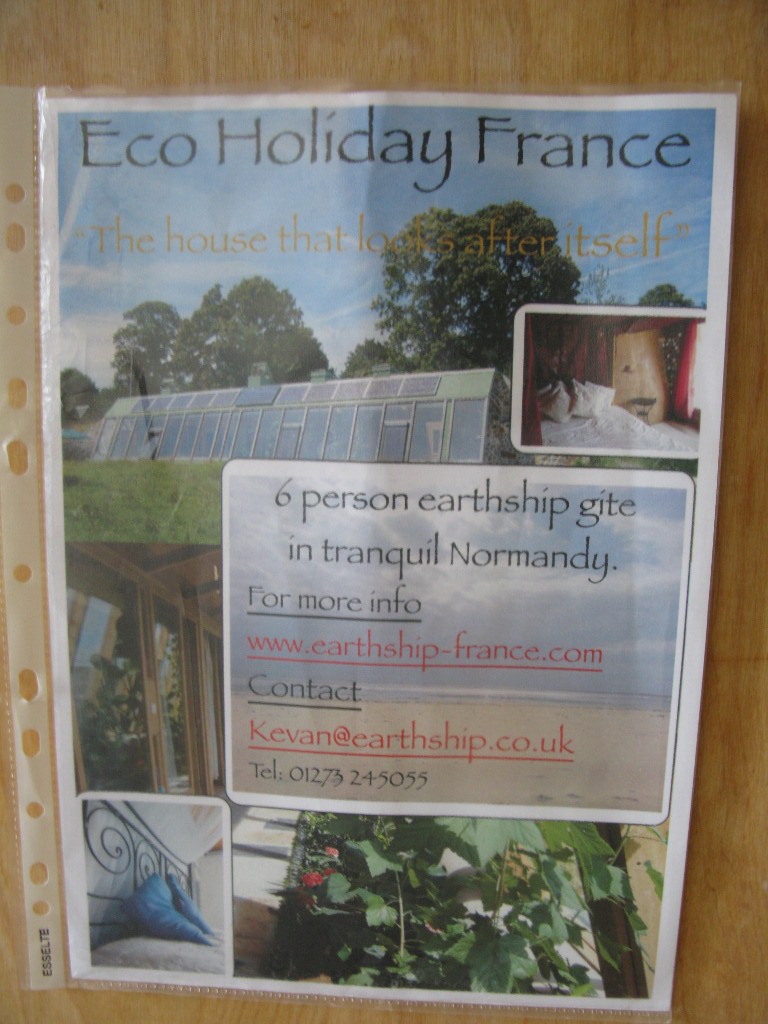A plastic-covered advertisement for a travel package is displayed on a wooden surface. The header reads "ECO HOLIDAY FRANCE" in bold black letters, subtitled by the phrase "The house that looks after itself" in yellow. Set against a backdrop of a blue sky with lush green trees, the central image features a greenhouse-like building with darkened windows. Below this, text announces a "six-person Earthship guide in tranquil Normandy," accompanied by multiple images of the home's interiors, including a cozy bedroom with white pillows and a brown-outlined cabinet, and a garden space. Contact details are also provided: for more information, visit www.earthship-france.com or contact kevin at earthship.co.uk, telephone 01-273-245-055.